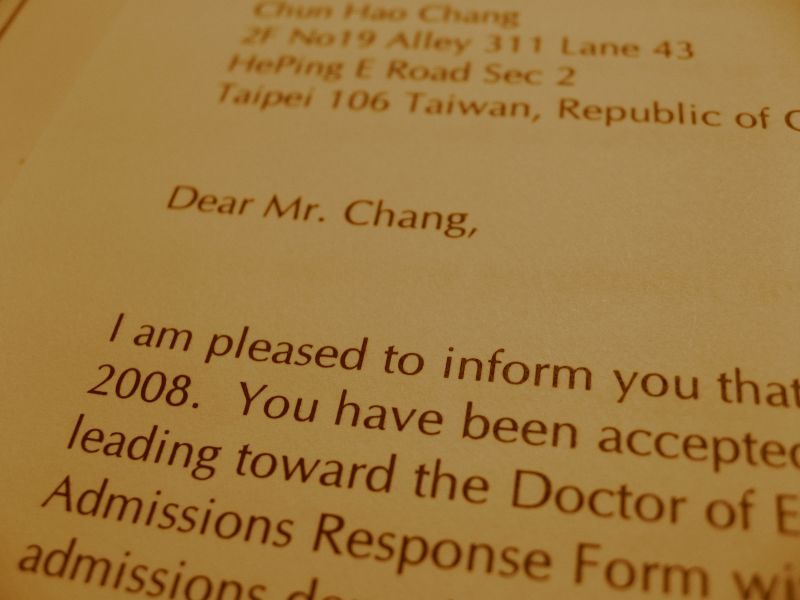The image features a photograph of a partially cut-off letter against a dark tan, light gold background. The paper looks aged, with dark brown or golden brown print. In the top left corner, there is a return address that reads:

Chan-Hao Chang,\
2F, No 19, Alley 311, Lane 43,\
He Ping E Road, Sec 2,\
Taipei 106,\
Taiwan, Republic of

Below the address, the letter begins with "Dear Mr. Chang," followed by a partially visible message. The legible portion reads: "I am pleased to inform you that..." before the text is cut off. Additionally, part of the letter mentions the year 2008 and something about an acceptance, but the right side of the text is truncated and unclear. The entire letter is positioned at a slight slant, making some parts difficult to read. Overall, the letter appears to be an old piece of correspondence.